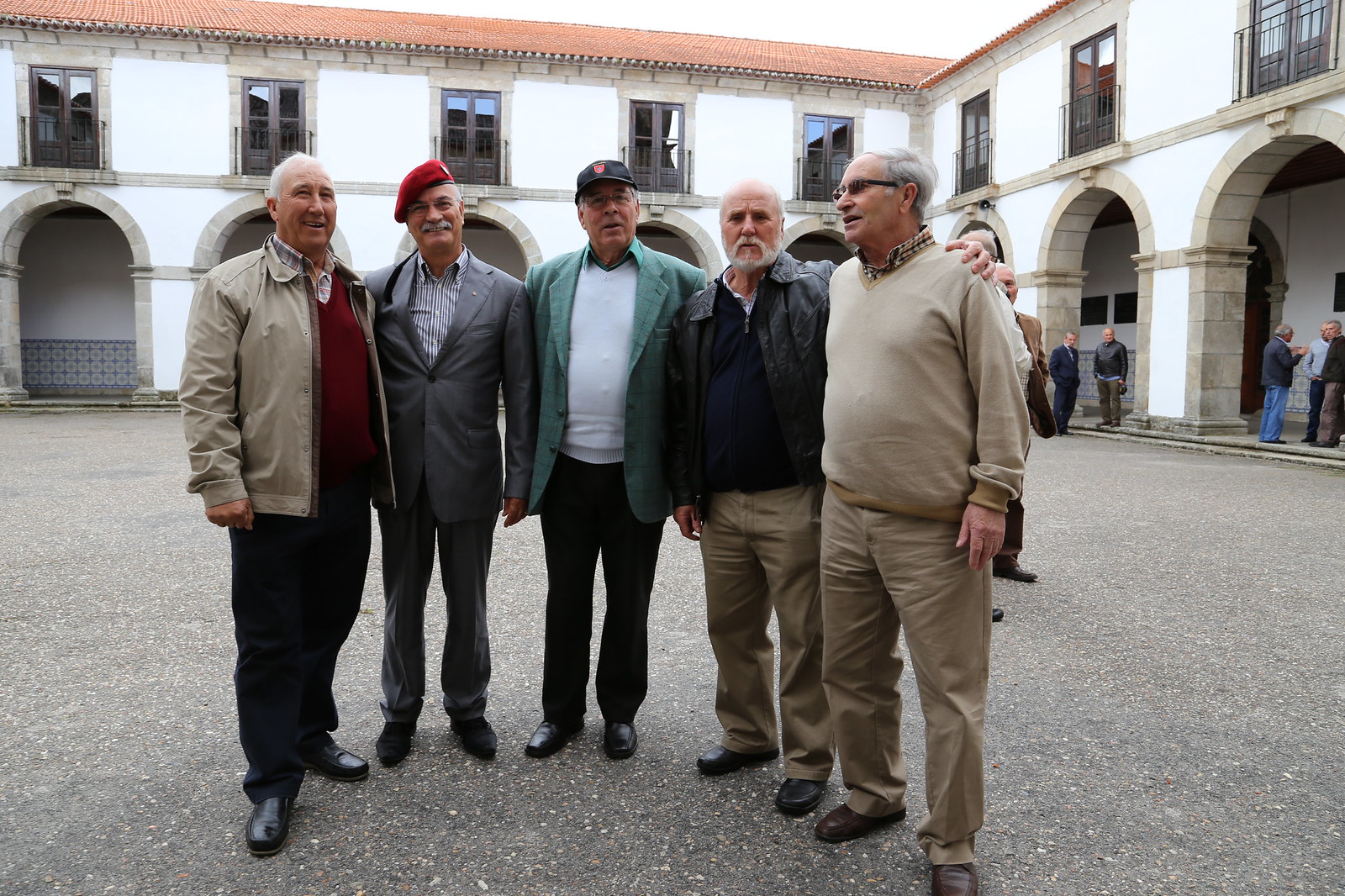In this detailed photograph, five elderly men, possibly in their 60s, are huddled together in a seemingly affectionate and convivial pose, perhaps indicating a reunion, possibly military. The men stand shoulder to shoulder, some with arms around each other, in a paved, gravelly gray courtyard. 

They are positioned in front of a building complex set at a right angle, featuring multiple black windows—five on the visible section on the left side and three on the right, with additional windows cut off by the frame. The building has a series of arches on the ground floor that serve as entryways, under which some people can be seen standing. The building consists of white walls with a sloped, triangular orange roof.

From left to right, the first man sports a tan short jacket over a red sweater, an open shirt, black pants, and has white hair. Next to him is a man in a buttoned gray suit with a checkered collared shirt and a striking red beret, accented by a mustache. Standing beside him, the third man wears a pale green-blue jacket over a white sweater, a dark baseball cap, and black pants. The fourth man is dressed in a black leather jacket, a dark blue sweater, and khaki pants, with his arm affectionately around the fifth man. The last man on the right wears a pale beige over-shirt over a checkered beige shirt and khaki pants, complemented by his glasses. They all appear relaxed and are facing forward towards the camera, with one man on the right slightly turned to the left.